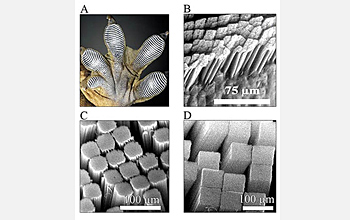The image is a composite of four black and white microscopic photographs arranged in a square, each labeled A, B, C, and D from top left to bottom right. The entire composite is bordered by a gray outer edge with a white inner border. 

- **Image A (top left)**: A highly magnified, round view of an organic structure, possibly showing bulb figures emerging from stems.
- **Image B (top right)**: Another microscopic view showing detailed linear structures with square-like tops. It includes the label "75 UM" beneath a prominent white bar.
- **Image C (bottom left)**: An overhead perspective showing numerous small square structures closely packed together. It features the label "100 UM" with a chunky white line beneath it.
- **Image D (bottom right)**: Similar to image C but with more defined, straight-edged square structures. It also includes the label "100 UM" with a chunky white line below.

Each image provides a different level of magnification and detail, focusing on varying aspects of what appears to be a microscopic study of an organic or biological sample.